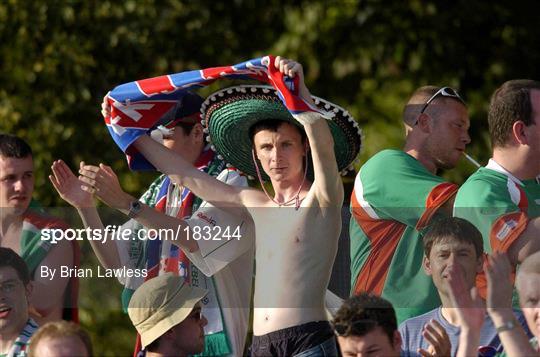In this vibrant outdoor photograph, a gathering of spectators, likely at a sporting event such as a soccer match, is captured with striking clarity. Central to the image is a shirtless, slender man donning a large, green-brimmed Mexican sombrero. He stands prominently, holding a blue and red striped banner with white delineations high above his head. His raised arms and the banner draw immediate attention. Surrounding him are numerous other spectators; some are clapping and others have their hands raised, all seemingly engrossed in the event. The crowd is dressed in colorful attire, with some individuals appearing to wear team colors, contributing to the festive atmosphere.

The sunlight illuminates the faces and bodies of the people, enhancing the vividness of the scene. At the bottom of the image, there is a gray transparent strip with white text that reads "sportsfile.com/183244 by Brian Lawless," indicating the photograph's source. The background is adorned with out-of-focus green foliage, providing a contrasting natural backdrop to the animated crowd. The combination of focused fans and blurred greenery adds depth to the image, making the central figures stand out even more.